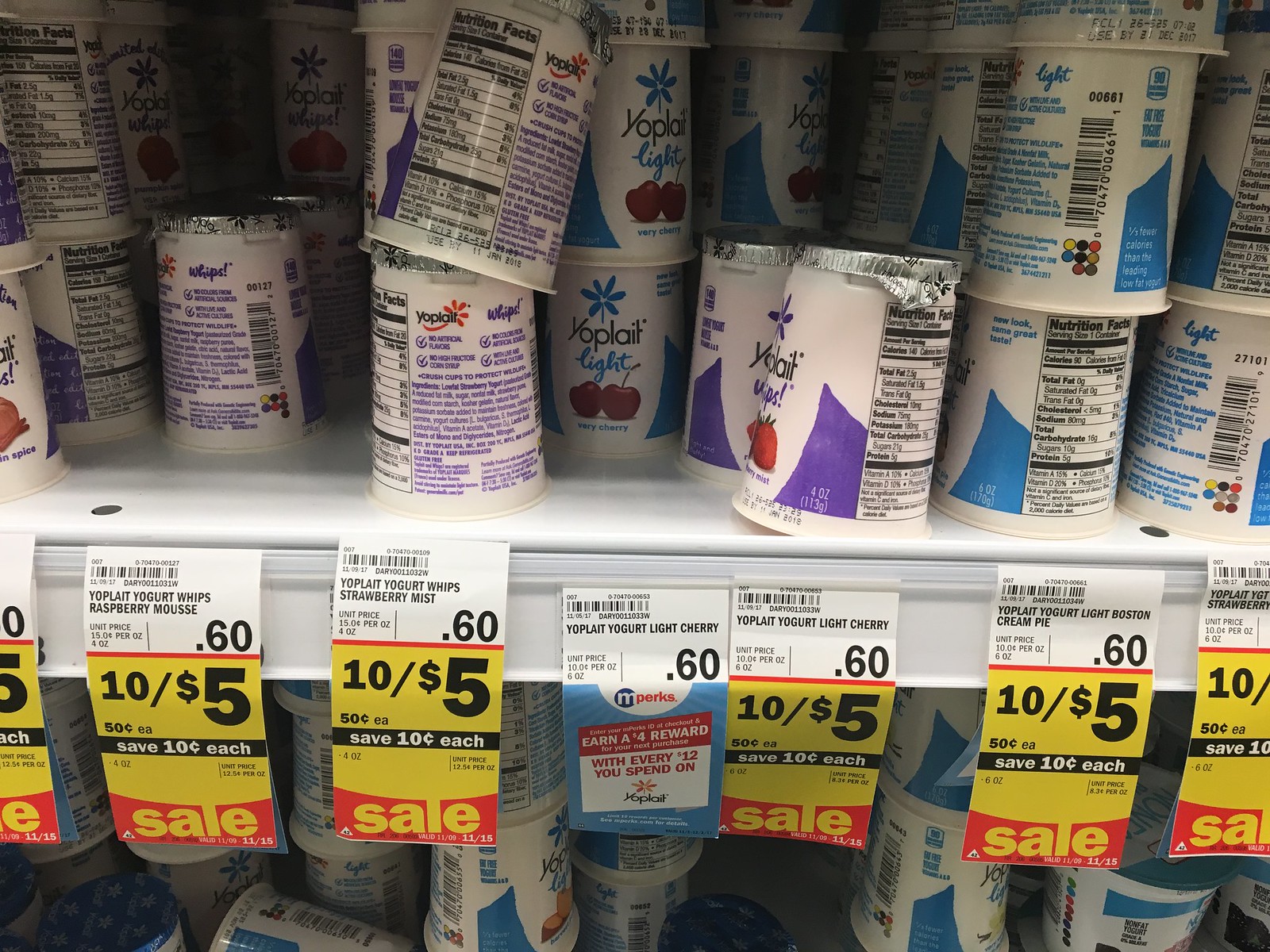This photograph captures a close-up view of a well-organized yogurt display in a grocery store. The shelves, which are white and located in a well-lit area, predominantly showcase various flavors of Yoplait yogurt. The yogurts have different labels, with common colors being purple, blue, white, and dark blue splotches. Each yogurt cup displays a distinctive Yoplait logo featuring a blue flower accompanied by the word "Yoplait" in black lettering, and below it, "light" written in blue cursive. Specifically, one of the flavors highlighted is "Very Cherry," adorned with an image of two cherries.

Beneath the yogurts, pricing and promotional signage are clearly visible. The price tags are primarily yellow with black numbers, indicating a sale price of $10 for 5 units, equivalent to 60 cents each. Additionally, there is a promotional coupon attached to the shelf, stating, "Earn a $4 reward with every $12 you spend," with "Yoplait" prominently noted at the bottom of this coupon. The visible tags and signs further detail specific yogurt varieties such as Yoplait Whips Raspberry Mousse, Yoplait Whips Strawberry Mist, and Yoplait Light Boston Cream Pie, all priced at $10 for 5.

The shelves also contain additional rows of yogurt stacked about three high. However, the contents on the lower shelf are less visibly detailed but appear to be more Yoplait yogurt products. Overall, this image illustrates a well-stocked and actively promoted Yoplait yogurt section within the store.